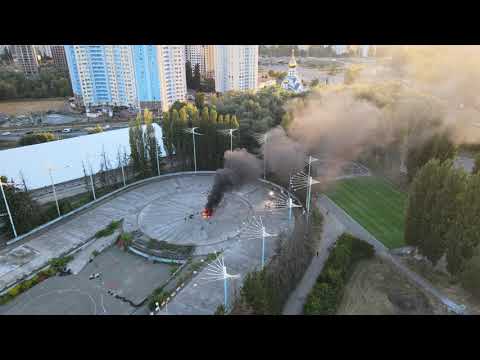This aerial image, taken during the day from a high vantage point, likely from a building or a helicopter, captures a dramatic scene of a fire erupting from a large, cylindrical, Coliseum-like sports stadium. The fire has breached the roof at the very center, sending thick, dark gray smoke billowing upwards, gradually lightening as it ascends but remaining dense throughout. Surrounding the stadium is a mix of urban and green spaces: high-rise buildings that resemble offices or hotels, a structure that appears to be a church with domed towers or possibly a mosque with golden domes, and a park-like field bordered by trees to the right. There are also roads and a highway visible, along with a parking lot in front of the stadium that is conspicuously devoid of any vehicles. The panoramic scope of the shot also hints at a distant body of water, possibly a river or bay, beyond the cityscape.